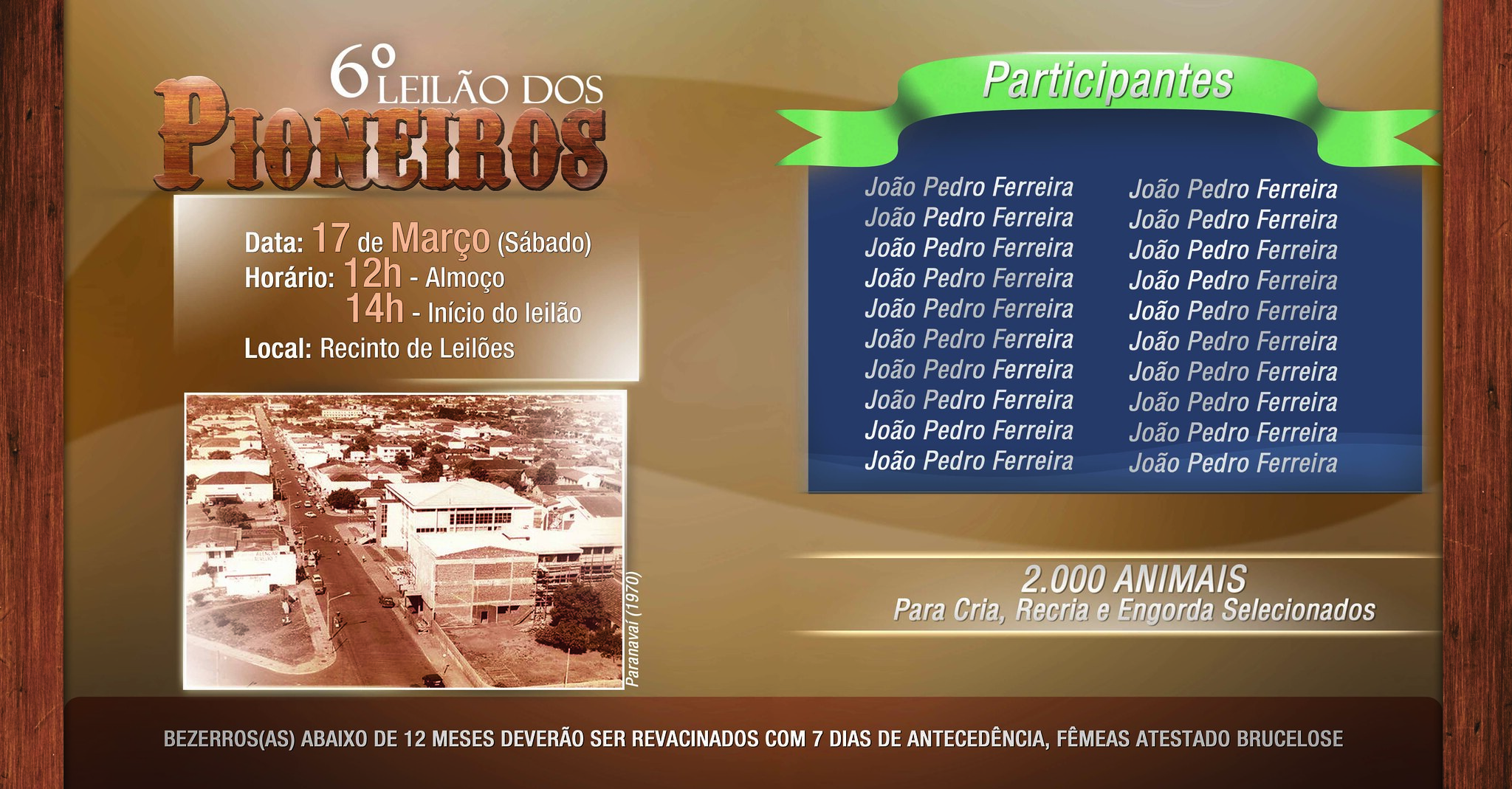The poster, likely an invitation or announcement, is framed with wood and presents a detailed layout in colors of green, blue, gold, and brown, complemented by white text. It is written in Portuguese and announces the 6th Leilão dos Pioneiros (Pioneers Auction). Key information includes the date, "17 de março," time, "horário 12h" (to 2 p.m. indicated as "14h"), and location, "Recinto de Leolos."

The background is predominantly tan with a golden-brown hue, with a brown frame going around the entire poster. On the left side, the event details, "data: 17 de março" and "horário: 12h - 14h," are clearly stated in white and orange text. A photograph, appearing to be a black and white image of a historical city or colony, is located on this side as well.

The right side features a green ribbon with a V-cut on either end, displaying the title "PARTICIPANTES" in white letters. Below this ribbon, two columns list names, primarily "João Pedro Ferreira," suggesting a repeated mention of a key participant. Additionally, the poster notes "2000 ANIMAIS," potentially highlighting the number of items or participants involved. Towards the bottom, there is a beige line with white lettering stating important reservation information, emphasizing that reservations must be made seven days in advance.